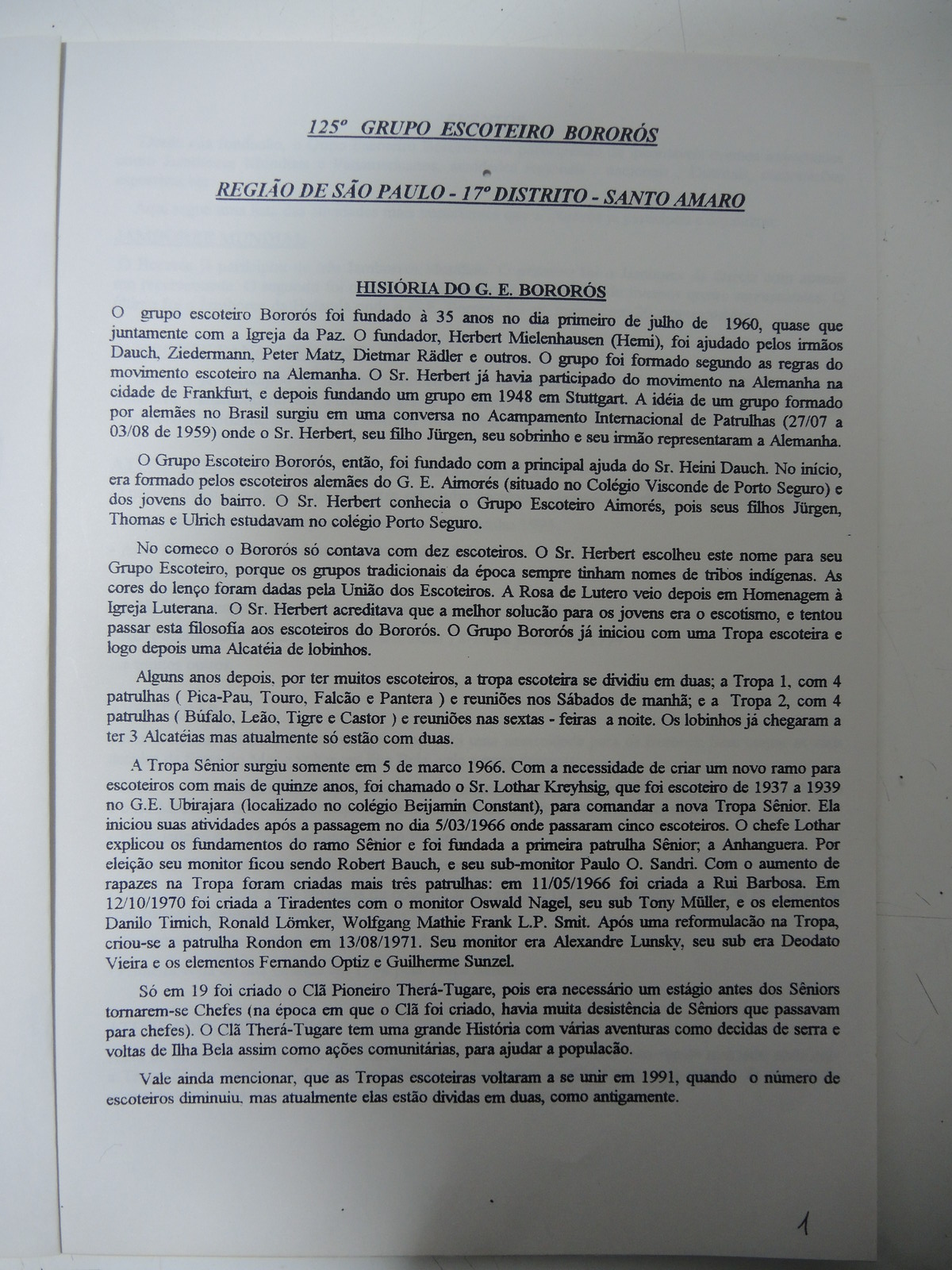This image captures a white sheet of paper lying on a similarly white background, which may be a table or another surface. The paper features black lettering in what appears to be Spanish. At the very top, the underlined and capitalized text reads "125 GRUPO ESCOTERO BOROROS." Below this, a second underlined title states "Regagio de Sao Paulo 17 Distrito Santo Amaro." A third underlined subtitle, "Historia do GE Bororos," introduces six to seven paragraphs of text. The paragraphs begin with "O Grupo Escotero Bororo full fundado 35 anos no dia primario," and continue in the same language. The paper also features a whimsical black number one in the right-hand corner, and the entire page is printed in a Times New Roman font. There is a soft shadow on the right half of the page, making the left side appear brighter.